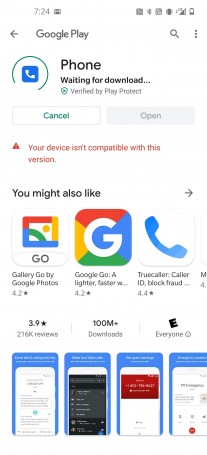The screenshot depicts a mobile device screen with the Google Play Store interface visible. The background is predominantly white. At the top, the text "Google Play" is displayed in black font, accompanied by a back arrow on the left. Below this header, a blue and white phone icon is enclosed within a broken green circle. To the right of this icon, the text reads "Phone - waiting for download" in black, followed by "Verified by Play Protect." A green "Cancel" button is located below this description, beside a grayed-out "Open" button.

This screen captures the status of the Phone app, which appears to be in the process of downloading. Near the bottom, a red warning rectangle is prominently featured, alongside a red alert triangle. The accompanying text states in red, "Your device isn't compatible with this version," signaling an issue with the app's compatibility with the device in use.